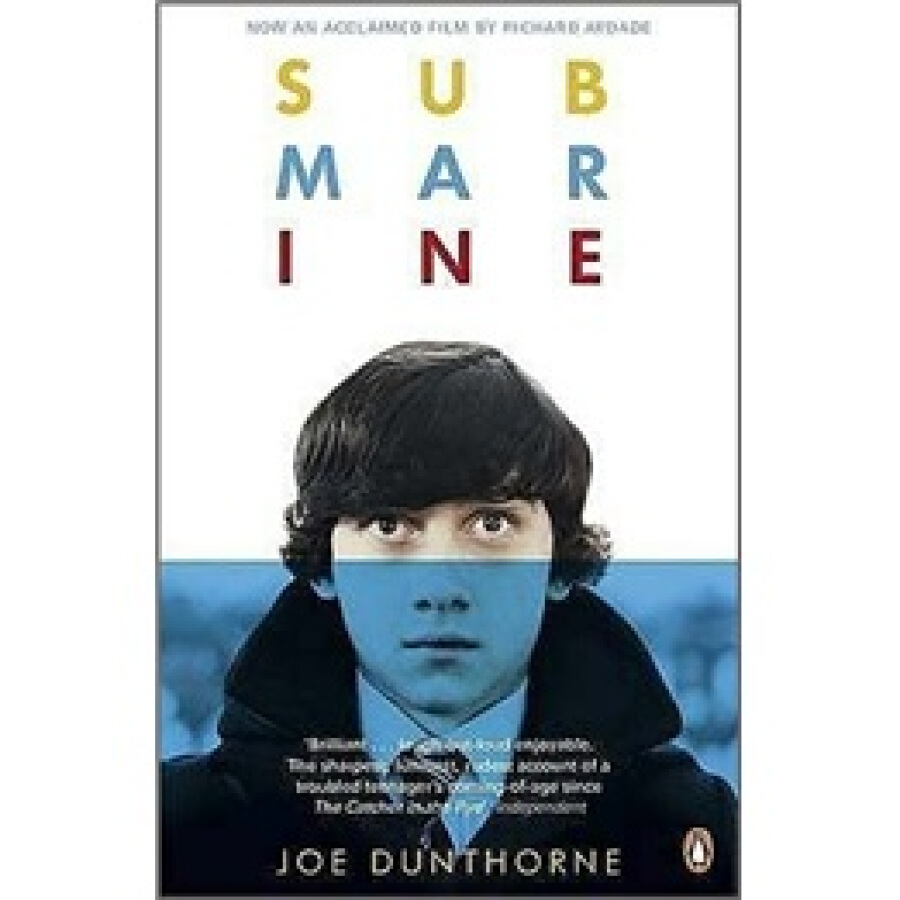The image depicts a movie poster for the film "Submarine," directed by Richard Ayoade. The title "Submarine" is stylized across three lines with "S-U-B" in yellow, "M-A-R" in teal blue, and "I-N-E" in maroon. A young boy with longer hair covering half of his ears, styled to curl out at the front, occupies the center of the poster. He is dressed in a jacket with the collar upturned, paired with a buttoned-down dress shirt and a tie. The upper half of his face is set against a white background, which gradually transitions to a blue background for the lower half, giving an impression of submersion. The boy's image fades from crisp to blurred towards the bottom. Above the title is the text "Now an acclaimed film by Richard Ayoade," though this is slightly blurred. At the very bottom, the name "Joe Dunthorne" is clearly visible in white letters. The poster features a palette of black, gray, white, yellow, light blue, red, and brown, with a slightly pixelated quality.